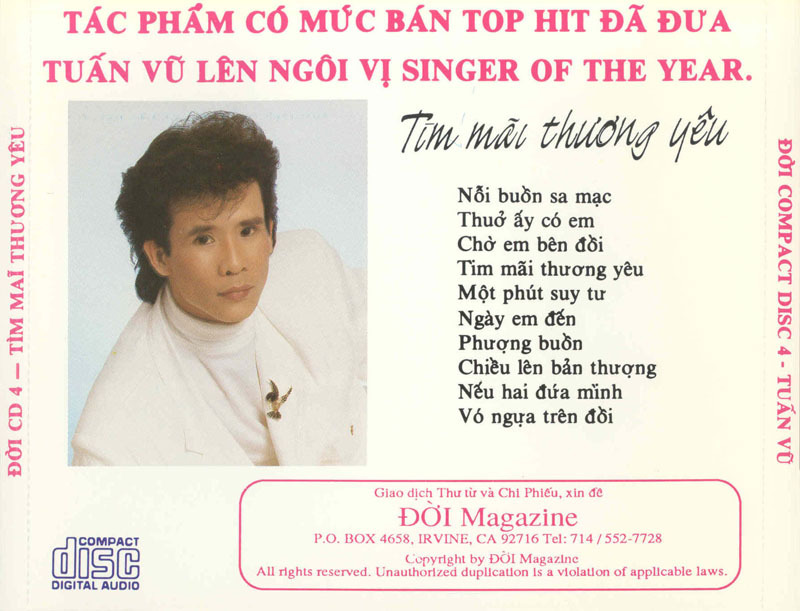The horizontal rectangular image is a poster predominantly featuring pink and black text, with a photograph of a male entertainer. At the top, there are two lines of large writing in pink, with only partial English phrases visible, such as "Top Hat" in the first line and "Singer of the Year" in the bottom line. Much of the text appears to be in Vietnamese. The center-left of the poster showcases a photograph of a man, presumably the "Singer of the Year," who appears to be Asian with puffy brown hair, wearing a white turtleneck adorned with a bird-shaped brooch. Below the photograph, "DOI Magazine" is written, followed by additional text. Toward the bottom right, a section contains the DOI Magazine address: PO Box 4658, Irving, CA 92716, and contact information; it also mentions copyright details. In the lower left corner, "Compact Disc Digital Audio" is printed, indicating the format of the entertainer’s work.